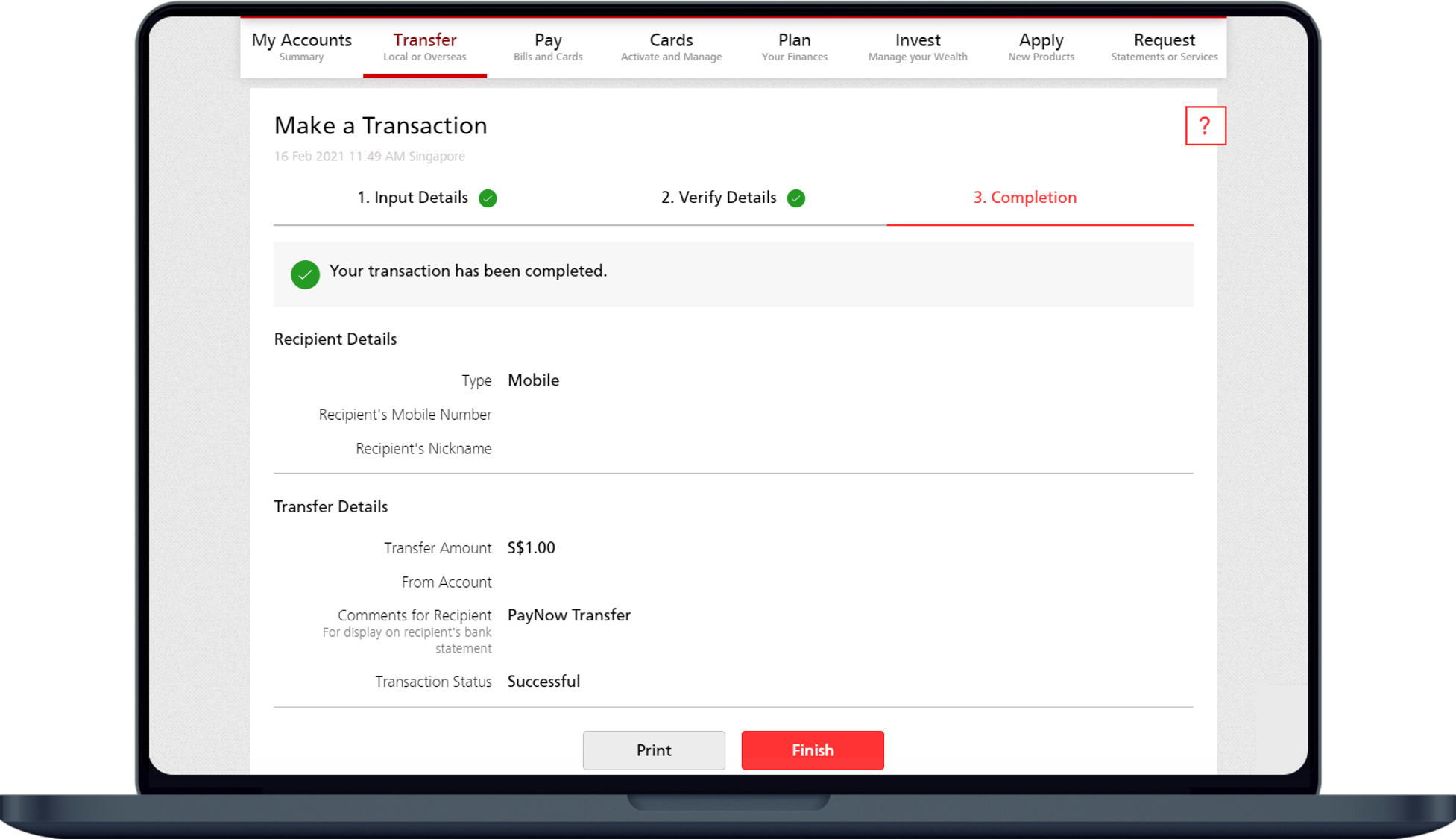The graphic depicts an open laptop screen with a minimalist white background. At the top of the screen, there is a navigation menu with various clickable links: "My Accounts," "Transfer" (highlighted in red), "Pay," "Cards," "Plan," "Invest," "Apply," and "Request," all written in black text. Directly beneath the selected "Transfer" option, a thick horizontal line underscores the word in red.

The main content of the screen features the title "Make a Transaction" in large black font. Beneath this, three sequential steps are listed: "Input Details," "Verify Details," and "Completion." The word "Completion" is prominently displayed in red and underlined. Below this header, a green circle with a white check mark signifies a successful transaction, accompanied by the bolded message, "Your transaction has been completed," written in black.

Further down, the screen provides two detailed sections: "Recipient Details" and "Transfer Details." These sections include various input fields and information, such as the amount transferred and selected options like "Pay Now" and "Transfer." The transaction status is clearly marked as "Successful" in bold black text.

At the bottom, two buttons are available for the user: a "Print" button with black text on a white background and a "Finish" button with white text on a red rectangular background.